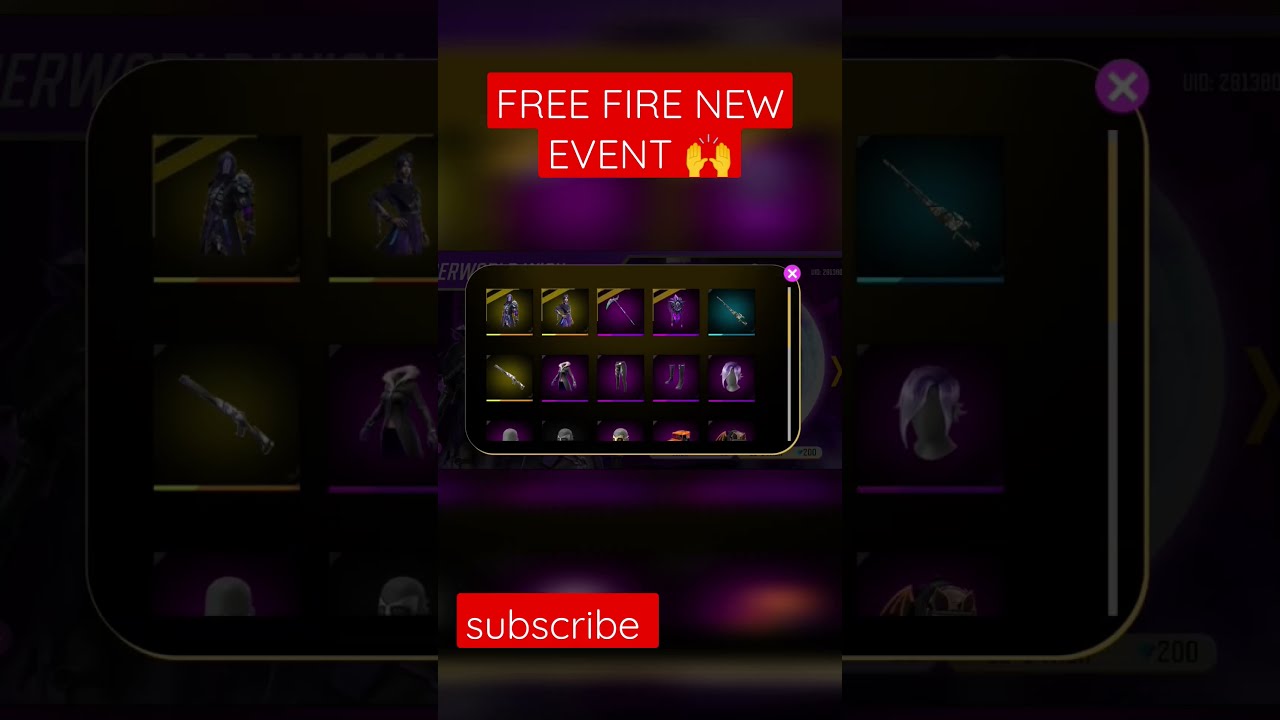In the image, a vertical screenshot showcases a dark-toned color illustration, heavily featuring purple, black, and yellow hues, with some turquoise accents. At the top of the screen, a red box with thin, all-cap white sans-serif text announces "FREE FIRE NEW EVENT," accompanied by an emoji of two raised hands with palms outward and thumbs facing each other. The background visually resembles a video game interface, suggesting a game inventory display with multiple selectable items in various colors including yellow, purple, and teal. On the top right of the interface, a purple circle with a white "X" acts as a close button. At the bottom of the image, another red box features the word "subscribe" in lowercase white text. The overall style is illustrative, hinting at a gaming event or update.